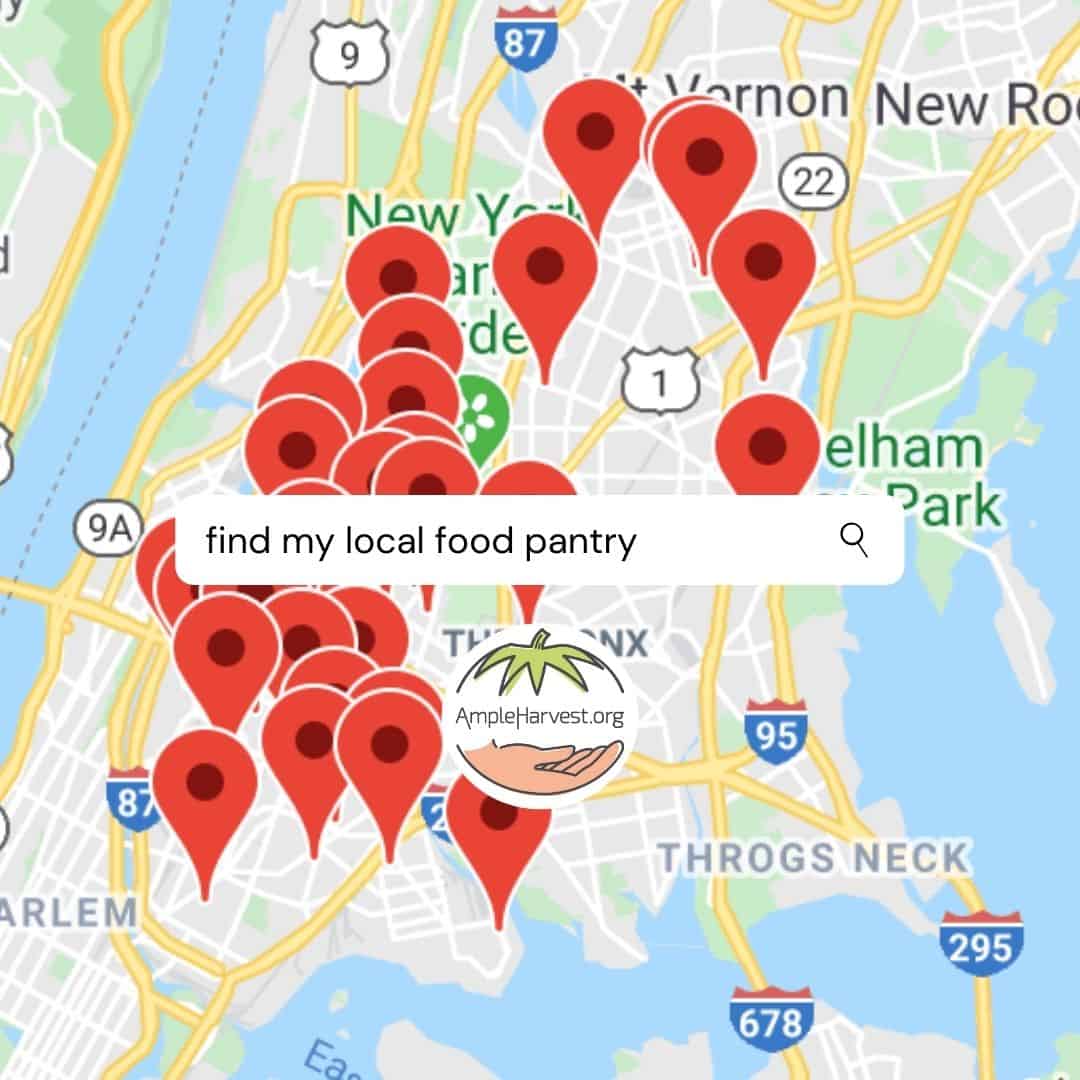This is a detailed screenshot of a map highlighting 32 red pins, each indicating different locations within New York. Various highways are clearly marked, including Highway 95, Highway 295, Highway 678, and Highway 87. The map also delineates both land and water features, as well as diverse areas such as Harlem. Parks and other significant regions are labeled, providing a wide-ranging overview of the city. The map features a prominent banner stating "Find My Local Food Pantry," and is sourced from AmpleHarvest.org, a platform dedicated to helping people locate food pantries.